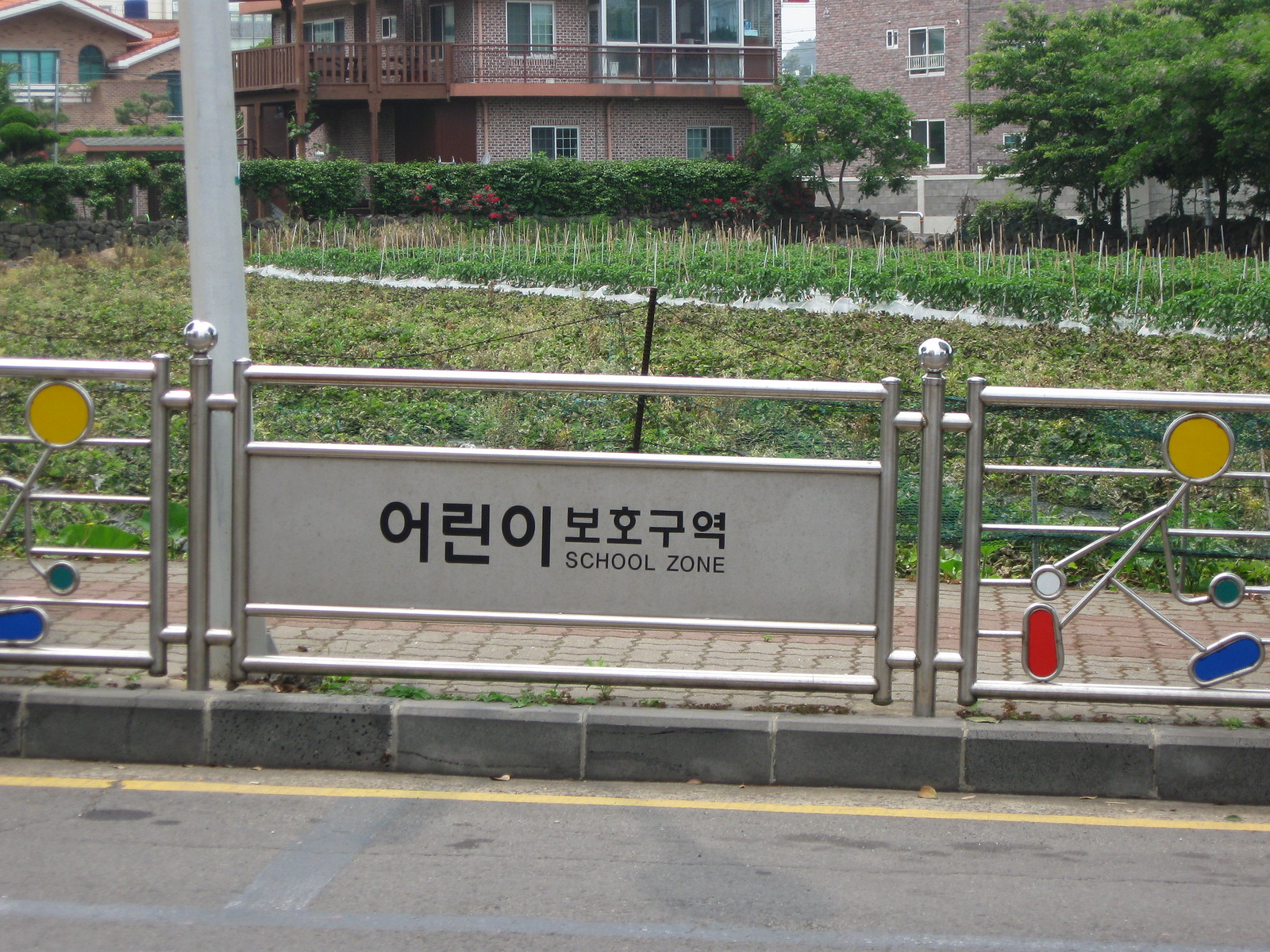This horizontally aligned rectangular image features a sign in front of a school. The foreground reveals part of the road with a yellow stripe on the edge, transitioning to a curb and a metal wire fence. The sign, affixed to the fence, includes black characters in an unidentified language, alongside the English phrase "school zone". The fence itself is adorned with colorful stick figure designs, suggesting children, composed of circular and oval shapes: a yellow circle for the head, white and green circles for the hands, and red and blue ovals for the feet. 

Beyond the fence lies a brick or cobblestone walkway, leading to a grassy area with tall weeds and scattered trees. The background features a brownstone building with multiple rectangular windows, though the picture's upper edge obscures the building's full height. No people are present in the image, and the scene is devoid of additional text beyond the posted sign.